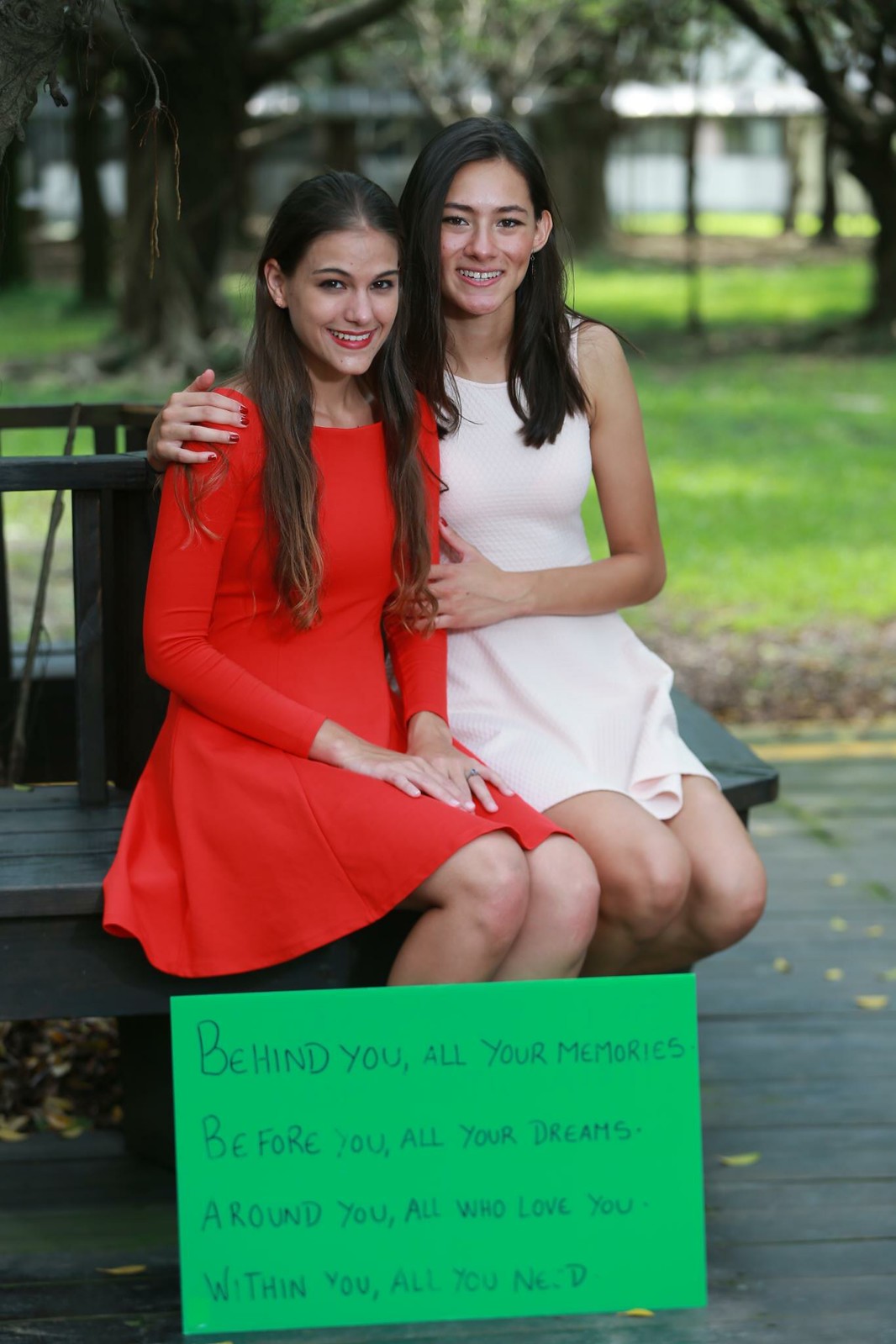In the picture, two young women with long, dark hair are sitting closely on a wooden bench in a serene, park-like setting. The woman on the left is wearing a red, long-sleeved dress that falls just above her knees, complementing her long, slightly wavy brown hair. She is smiling warmly at the camera with red lipstick and a happy expression. The woman beside her, on the right, is dressed in a white, sleeveless dress of similar length. Her darker black hair cascades down as she smiles gently, her right arm lovingly draped around the shoulder of the woman in red.

In front of their feet is a green rectangular sign with an inspiring handwritten message in bluish lettering: "Behind you, all your memories. Before you, all your dreams. Around you, all who love you. Within you, all you need." They seem to be alone in the peaceful park, surrounded by lush grass and trees, making it evident that they are sharing a tender moment together. Their joyful expressions and close posture suggest a deep bond, possibly hinting that they are sisters. The background is devoid of other people, focusing the scene purely on their connection and the tranquil environment.